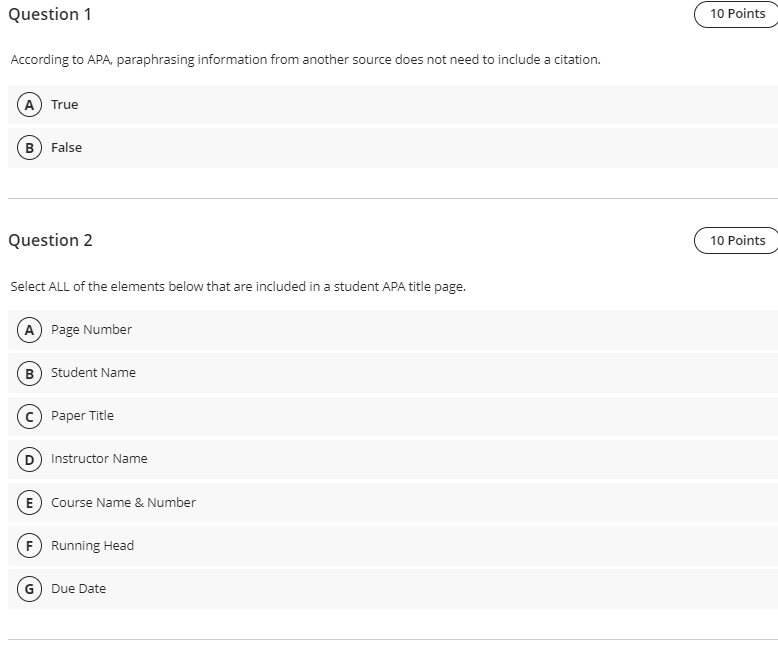A cropped screenshot of a web page is displayed, with the right-hand side and top portions cut off. The visible segment starts with a header labeled "Question 1." The screen shows text stating, "According to the APA, paraphrasing information from another source does not require a citation." This appears to be part of a test or quiz format, as indicated by a partially visible oval button on the right-hand side that reads "10 points" in bold, black text with a black border around it. 

Below this header, there are two answer options: "A. True" and "B. False," both set against gray rectangles that span the width of the screen.

Following this, "Question 2" is presented, also valued at 10 points. It asks the participant to "Select ALL of the elements below that are included in a student APA title page." The options, listed in gray rectangles with small white gaps between each, are:
- A. Page number
- B. Student name
- C. Paper title
- D. Instructor name
- E. Course name and number
- F. Running head
- G. Due date

A black line separates the two questions, and another black line is located at the bottom of the visible portion of the screenshot.